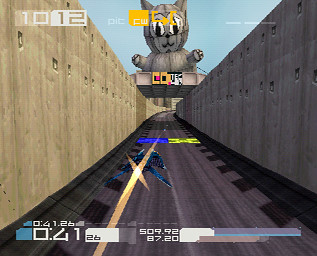This is a detailed screenshot from a futuristic racing video game, designed for play on either computer or console. In this captivating scene, a small, blue spaceship is racing through winding tunnels framed by concrete walls and a dirt-like track, hovering slightly above the ground. The spaceship is maneuvering skillfully through the course, adding a sense of speed and agility to the visual. Towering above the track, perched on the concrete barriers, is an enormous, three-dimensional statue of a cat, its presence both majestic and surreal. The sky in the background is a clear, vivid blue, adding a serene contrast to the intensity of the race. Additionally, on-screen elements display essential gaming statistics such as time and speed, framing the bottom and top edges of the image, providing players with real-time information crucial for navigating the course.